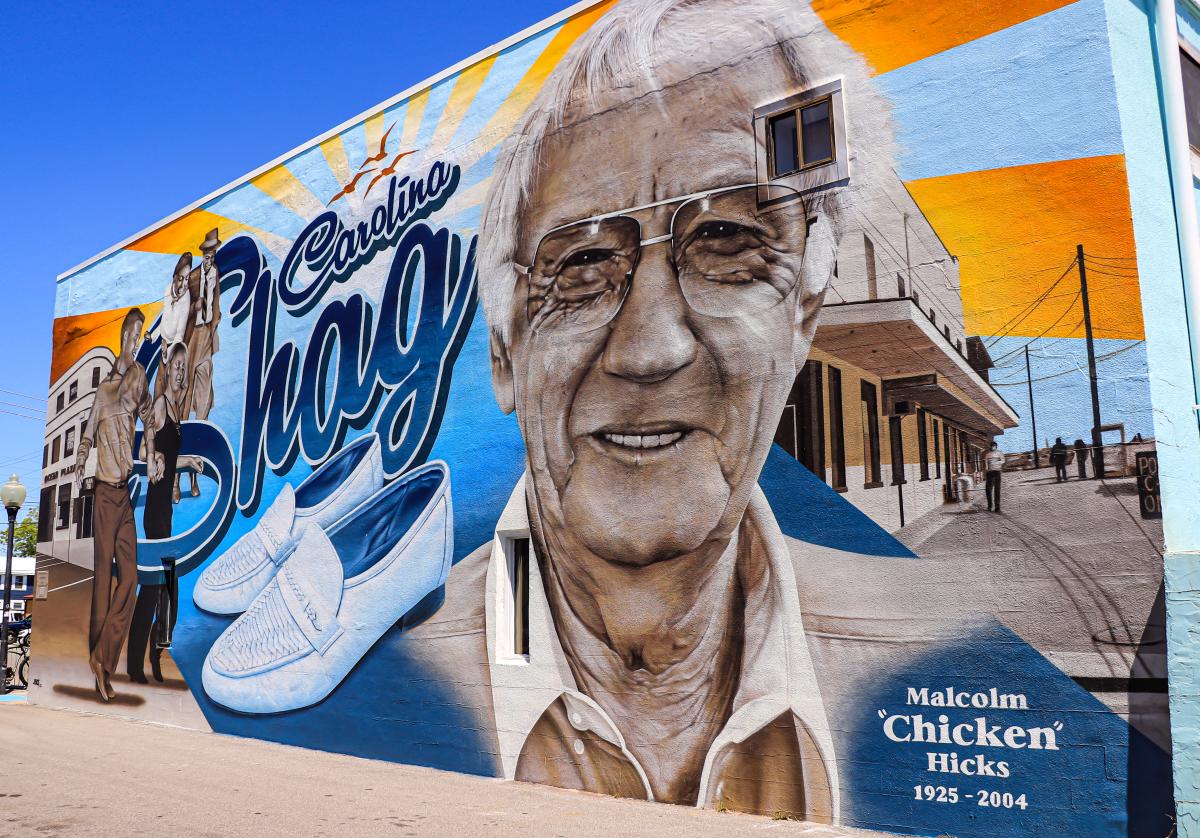The mural depicted in the image is painted on the side of a concrete building under a clear blue sky, adjacent to a lamppost. This colorful, rectangular mural commemorates Malcolm "Chicken" Hicks (1925-2004). Centrally featured, the mural portrays an old, gray-haired man with a smiling demeanor, wearing wire-framed glasses and a collared polo shirt. His nickname, "Chicken," is placed in quotation marks beside his full name at the bottom right, with the dates marking his life span.

To the right of Malcolm's portrait is a picture of an empty downtown street with a few figures walking, giving a sense of calm and nostalgia. The middle section above Malcolm showcases a vibrant blue cursive text reading "Carolina Shag," outlined in white. This text is set against a backdrop of yellow sun rays, accompanied by three seagulls circling above. Beneath this title, there is a pair of white leather loafers, symbolizing the dance style. 

On the left side of the mural, two couples are walking, captured in a black-and-white, old-fashioned photographic style, adding depth and historical context to the artwork. The overall composition presents a harmonious blend of elements, each highlighting different aspects of Malcolm Chicken Hicks's life and the cultural essence of the "Carolina Shag."